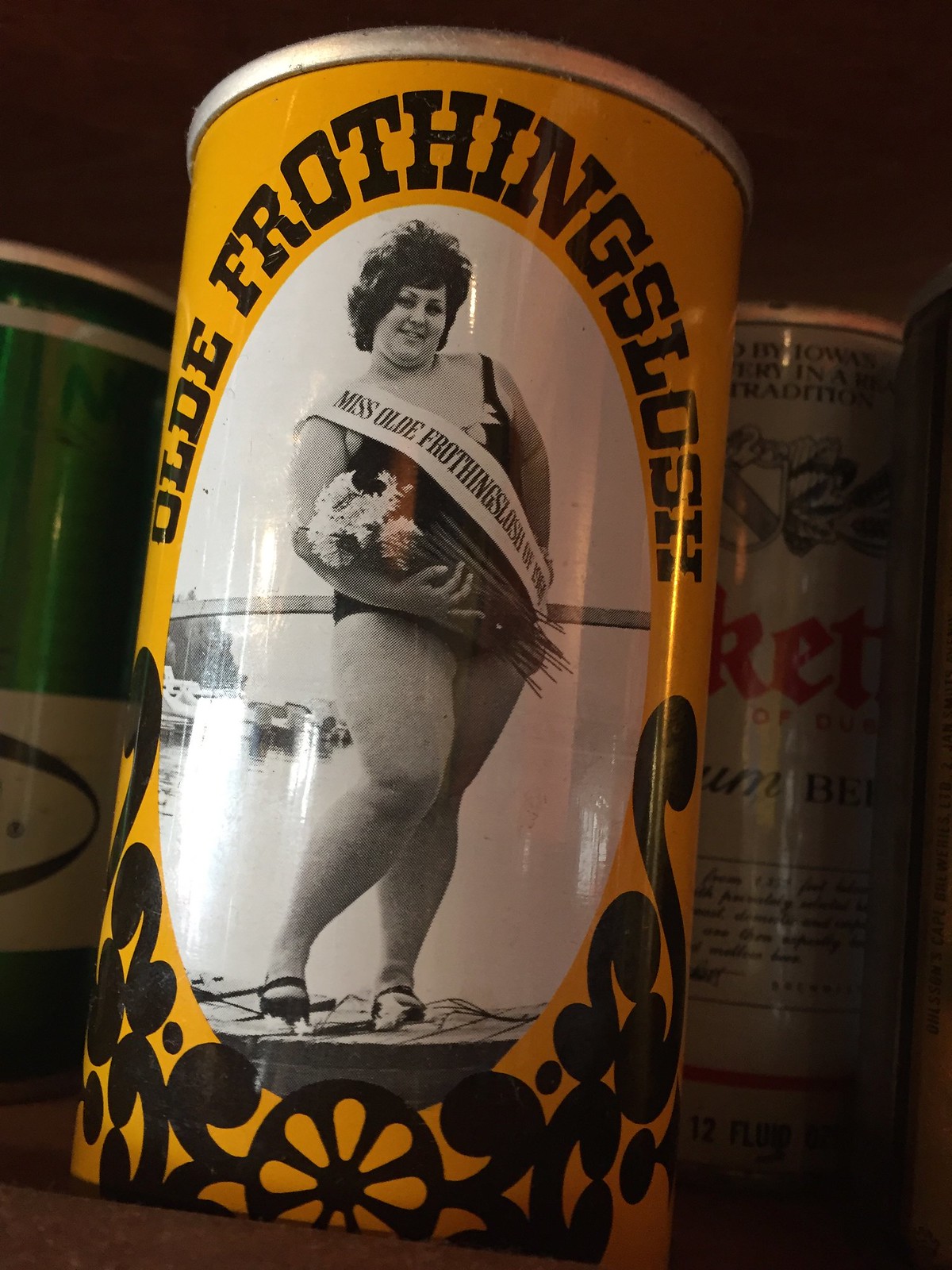This is a close-up photograph of a rectangular can in portrait orientation. The can prominently features the words "Olde Frothing Slosh" in black text set against a vibrant yellow background. A decorative black floral pattern adorns the bottom of the can. Centrally placed on the can is an oval, also in portrait view, containing a black-and-white photo of a woman in a swimsuit holding a bouquet of flowers. She is wearing a sash that reads "Miss Olde Frothing Slosh." In the blurred background, two other cans are visible; the one on the left is green, and the one on the right is silver.